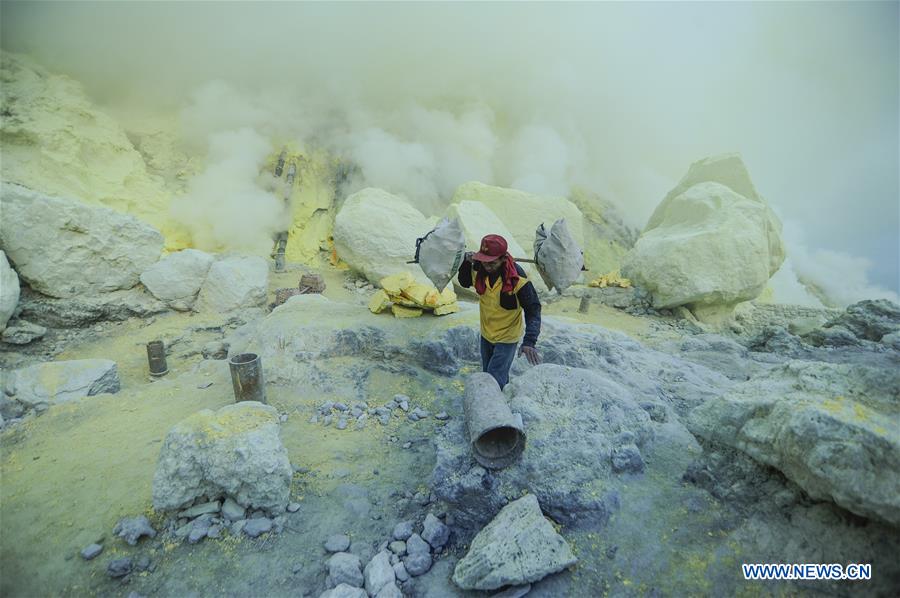This photograph, sourced from www.news.cn, captures a stark and rough outdoor landscape, possibly a mining area, characterized by an abundance of jagged rocks that dominate both the foreground and background. The rocks, mostly white with patches of yellow material, create a rugged terrain. Amidst this rocky expanse stands a singular figure, a man fully visible except for his knees, which are obscured by the surrounding rocks. He wears a red baseball cap with a bandana trailing down his neck, a distinctive yellow jacket with black sleeves — which might be a vest layered over a black jacket — and dark-colored pants, possibly black or dark gray. His right hand grips the top of his cap while his left hand extends outward, suggesting motion as he navigates the uneven ground. A tool or an item rests across his shoulder, though its exact nature remains unclear. Adding to the dramatic atmosphere, a thick pall of white to pale yellow smoke or dust billows in the background, further shrouding the distant view. The overall image quality is relatively good, rendering a vivid, detailed portrait of a harsh, desolate environment.